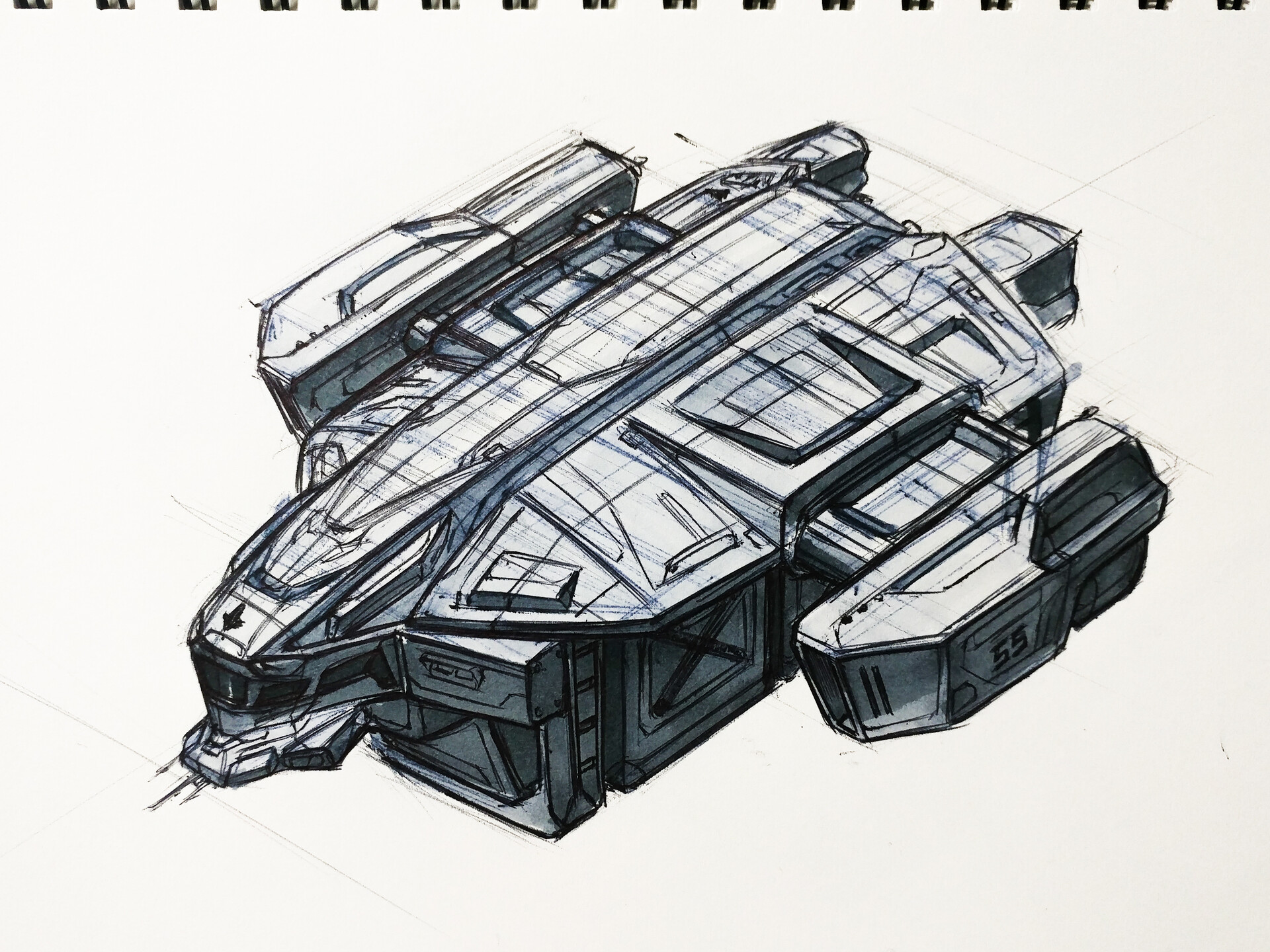The image is a detailed, hand-drawn sketch of an advanced, flat and rectangular-shaped blue spacecraft, depicted on a completely white background. The spacecraft, which resembles a space cargo ship, has a tapered face pointing towards the bottom left corner of the image. The sketch includes numerous panels, attachments, and jet-like features that lend it a geometric complexity, characterized by sketch lines illustrating its structure. At the bottom, two prominent rectangular shapes are pointing towards the top right corner. Notable markings include a section that appears to have windows along the left side and an 'X' and the number '59' on the far right side of the spacecraft. The overall design is intricate, though it seems to have been rendered in a somewhat hurried fashion, with hints of black accentuating various parts of the ship. The upper part of the image is bordered with a dotted black line, and the style and setting suggest a science fiction theme.